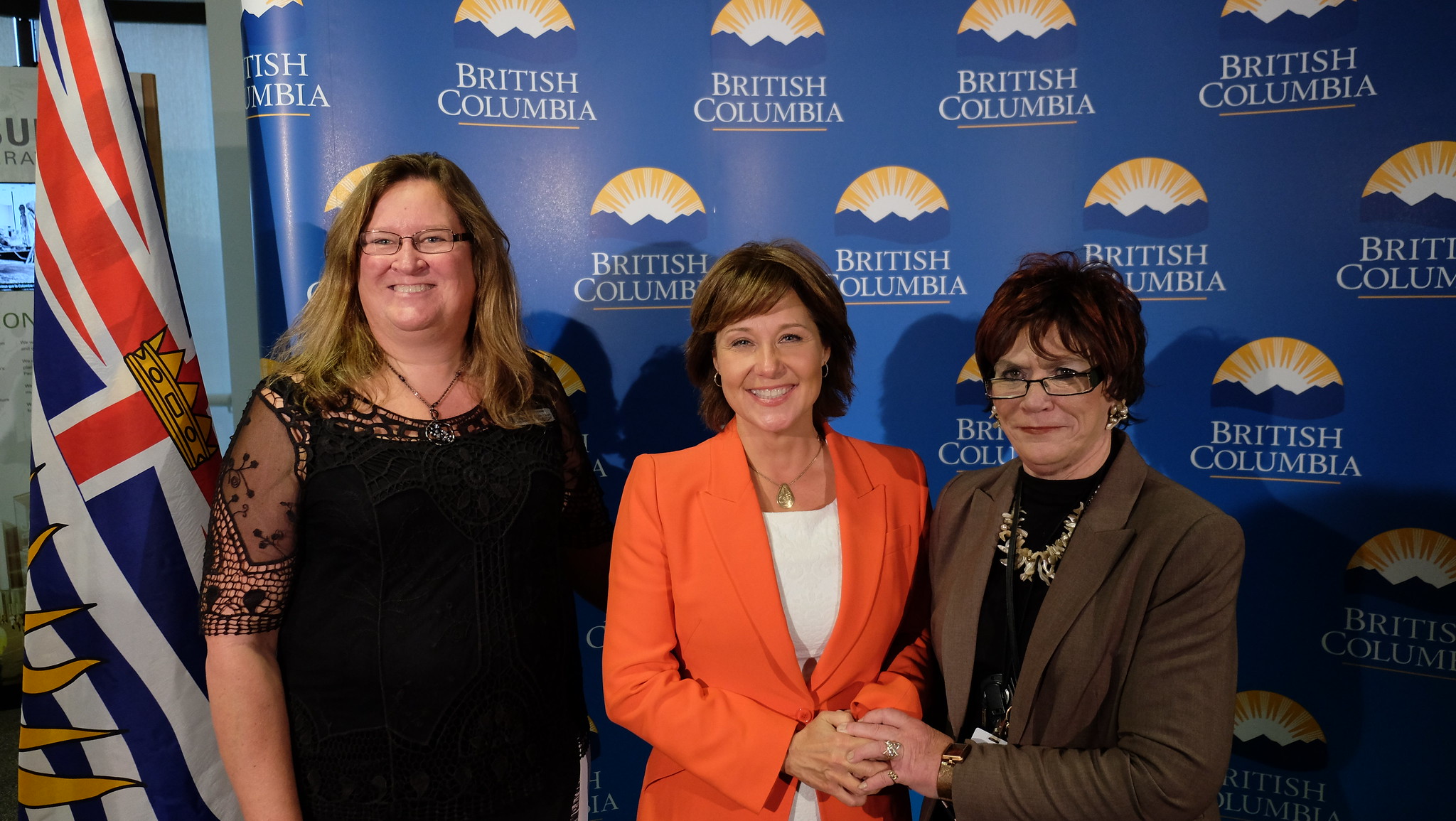This is a picture of three women standing in front of a large blue banner prominently displaying the British Columbia logo, comprising red, white, and blue elements with a semi-circle in yellow and a white underside on several symbols seen across the top, center, and bottom of the banner. To the left of the photo is the flag of British Columbia, featuring red stripes over a blue and white background with a gold crown. 

The woman on the left is dressed in a long black dress with transparent sheer sleeves and square glasses. She has long blonde hair and is smiling at the camera. The woman in the center, who is slightly shorter, wears an orange jacket over a white blouse, accessorized with a gold necklace. She has shoulder-length brown hair with bangs and is also smiling. She clasps the right hand of the woman to her left. The third woman, standing on the right, is clad in a brown jacket with a black blouse and a gold necklace. She sports short, reddish-black hair and black-framed glasses. Her left hand clasps the hand of the woman in the orange jacket, completing a touching gesture of camaraderie.